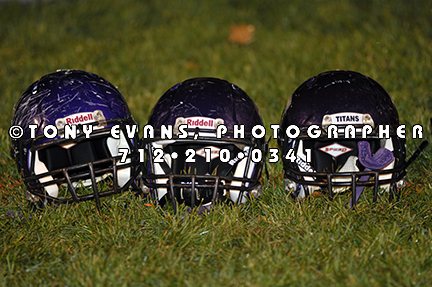The image is a landscape-oriented, color photograph depicting three American football helmets resting on slightly darkened, possibly autumnal grass. The helmets are predominantly purple with dark brown or dark purple face guards and white interior linings. They are aligned side-by-side on the turf, though not perfectly parallel, adding a natural variation to their positioning. The photograph's quality is modest, suggesting it might be a smaller, lower-resolution image. The scene appears to be dimly lit, possibly taken in the evening or under inadequate artificial lighting. Above the helmets, an orange, out-of-focus splotch, possibly a flower, can be seen in the top middle right-hand side of the image. Overlaying the photograph in bold white text is the copyright notice: "(C) Tony Evans, Photographer" followed by the phone number "712-210-0341." Additionally, the helmets feature the brand name "Riddell" and the team name "Titans" marked on them.